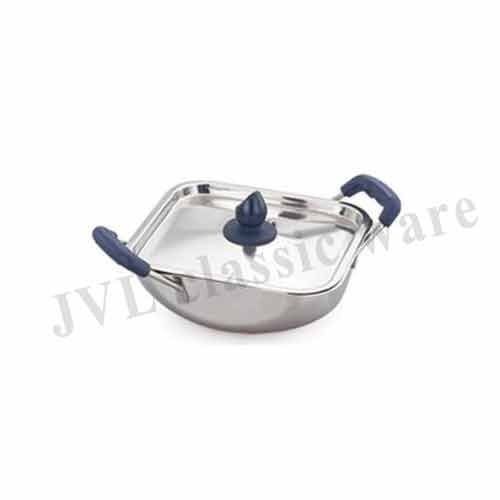The image depicts a square-shaped stainless steel cookware with curved edges, commonly referred to as a Kaday in Indian cuisine, ideal for serving rather than baking. The cookware features a stainless steel body with two metal handles that have black plastic coverings for heat protection. The lid is similarly made of stainless steel, equipped with a central black knob for easy lifting. The cookware's clean design is accentuated by a white background, with the brand name "JVL Classic Ware" prominently displayed in gray letters across the image. There are no other objects or furnishings visible, which maintains the focus on the elegant and functional cooking utensil.